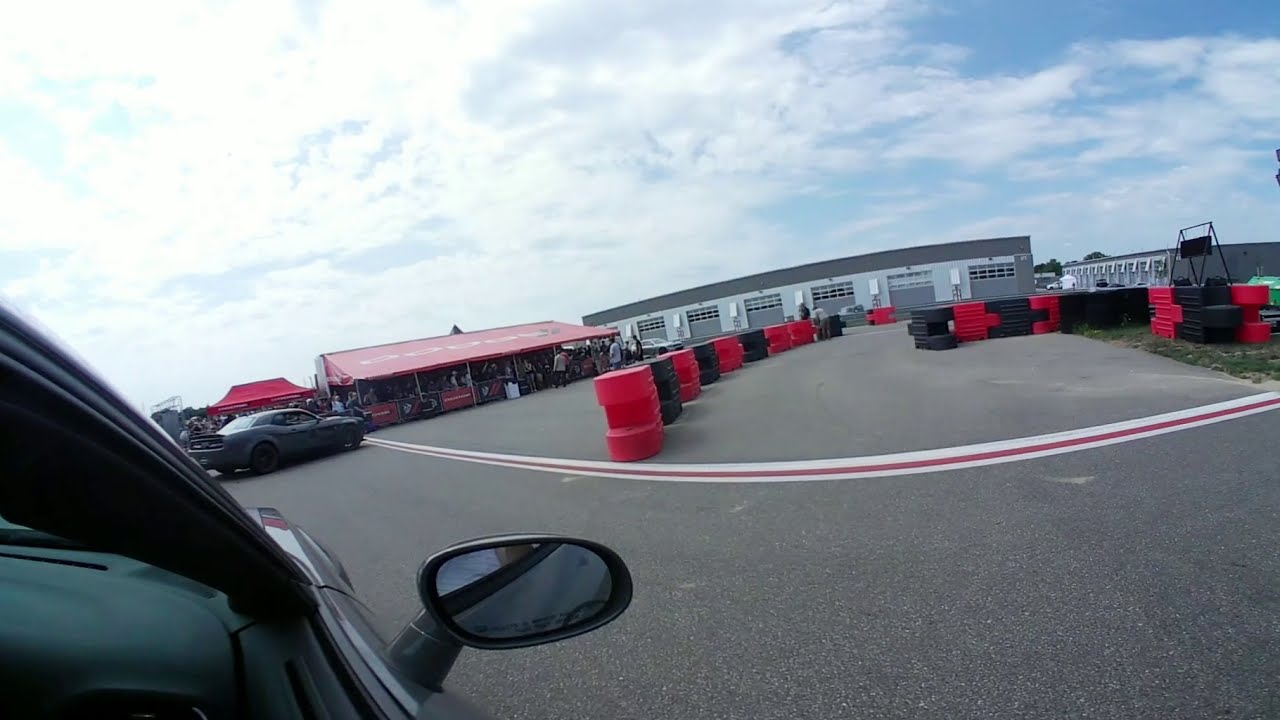Captured from the passenger side of a car window, this detailed photograph showcases a vast paved asphalt area stretching into the distance. Dominating the scene are stacks of alternating red and black tires, meticulously arranged in patterns that form barriers or curves leading towards a long gray warehouse with seven large, dark-gray bay doors in the background. To the left, a vivid red building or tent with an awning stands, occupied by several people and a parked dark gray Dodge Charger. Additionally, more tire stacks extend to the right, even spilling into the grassy areas beyond the pavement. The close-up perspective from inside the car reveals the dashboard and passenger-side rearview mirror in the bottom left corner. Overhead, the sky is dotted with puffy clouds and occasional blue patches, indicating a partly cloudy day.